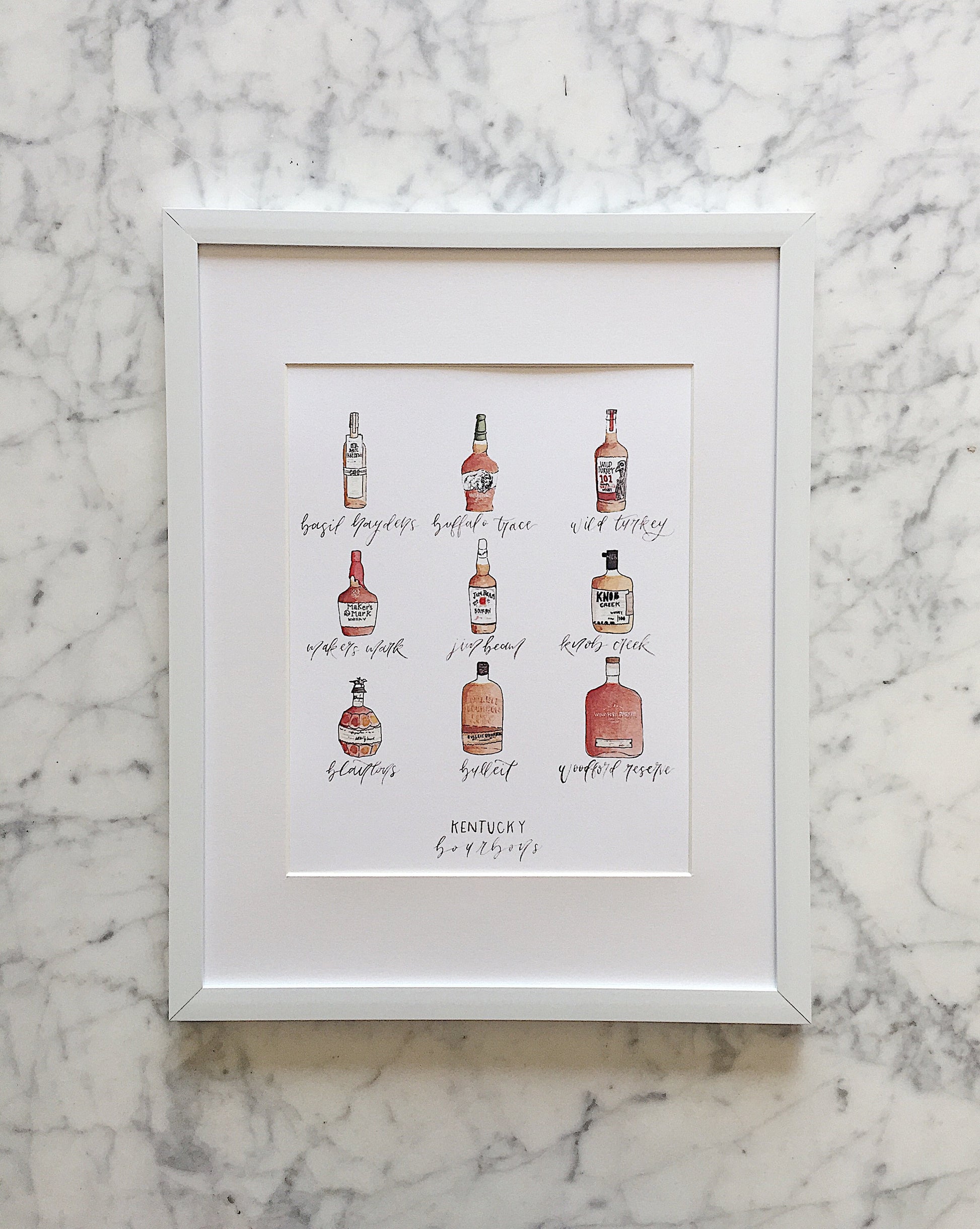The image depicts a detailed art piece, likely a watercolor drawing, of nine different Kentucky bourbon bottles. The bottles are arranged in a 3x3 grid within a white frame that also includes a white mat border. The background of the frame is a gray and white marble wall with black cracks. Below each bottle, in cursive writing, are the names of the bourbons, including recognizable brands like Maker's Mark, Buffalo Trace, Wild Turkey, Jim Beam, Knob Creek, and Bulleit. The artwork features a variety of bottle shapes and sizes, with some bottles having distinctive dark red or brown colors, indicative of the bourbon inside. The bottom of the image prominently features the inscription "Kentucky Bourbons" in elegant cursive handwriting.